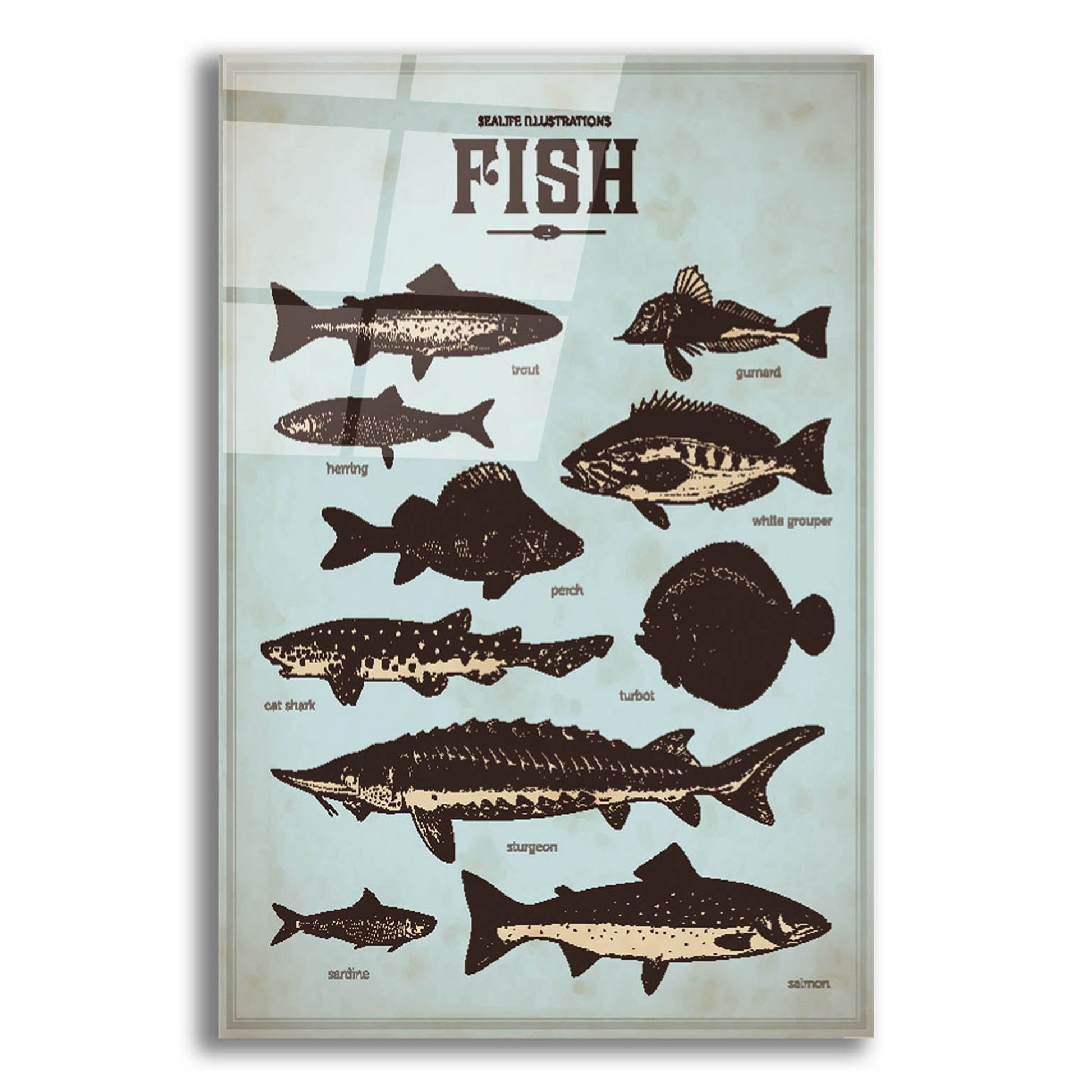The image is a detailed and reflective poster titled "Sea Life Illustrations - FISH" by Seattle Illustrations, featuring various fish species. The poster has a gray background with beige patches and is protected by a glass panel that reflects a window. At the top, in bold brown text, it reads "Sea Life Illustrations" and "FISH". The poster displays ten fish illustrations, labeled and colored in shaded brown, black, and tan. The fish are arranged in a chart-like manner, facing both left and right, against a distressed blue background with a gray border. From left to right, the fish include a trout, herring, perch, cat shark, sturgeon, sardine, gurnard, white grouper, turbot, and salmon. The largest fish, a sturgeon and a salmon, are prominently featured at the bottom, with the salmon extending across much of the right bottom corner. The poster presents a minimalistic yet detailed depiction of sea life, with small fish like sardine and herring, and larger ones such as the sturgeon and salmon, in dark brown and beige tones.